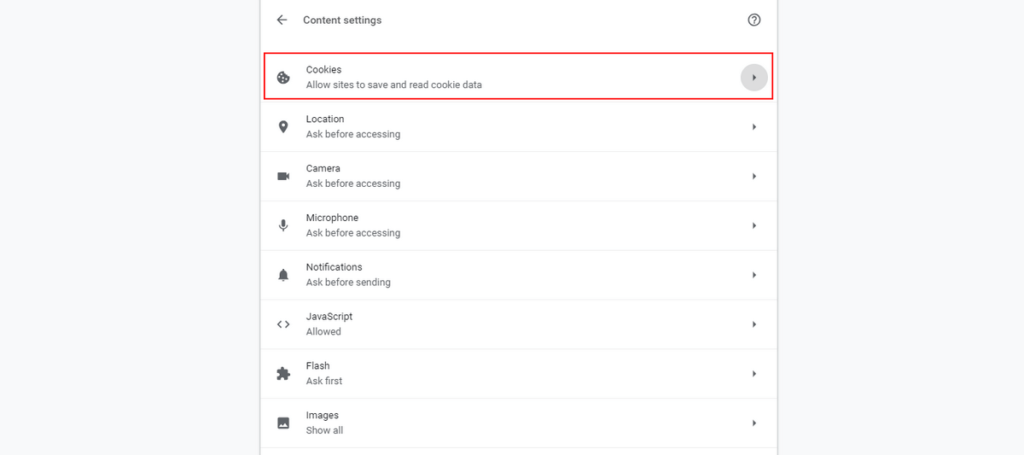This image displays a detailed view of a "Content Settings" window within a digital interface. The "Content Settings" heading is positioned on the upper left side, slightly indented from the screen's edge. To the left of the heading, there is a back arrow separated by a space. On the far-right side of the header, there is a circular icon with a gray outline and a white background, containing a gray question mark.

Below the heading, there is a listed menu comprising eight items. The first item is highlighted with a red square and is labeled "Cookies." Beneath the label, the description reads, "Allow sites to save and read cookie data." Adjacent to this description is an icon of a cookie with a quarter bitten off from the top right. Completing the layout, a gray right-pointing arrow is displayed on the far right of the "Cookies" item, aligning towards the screen's edge.